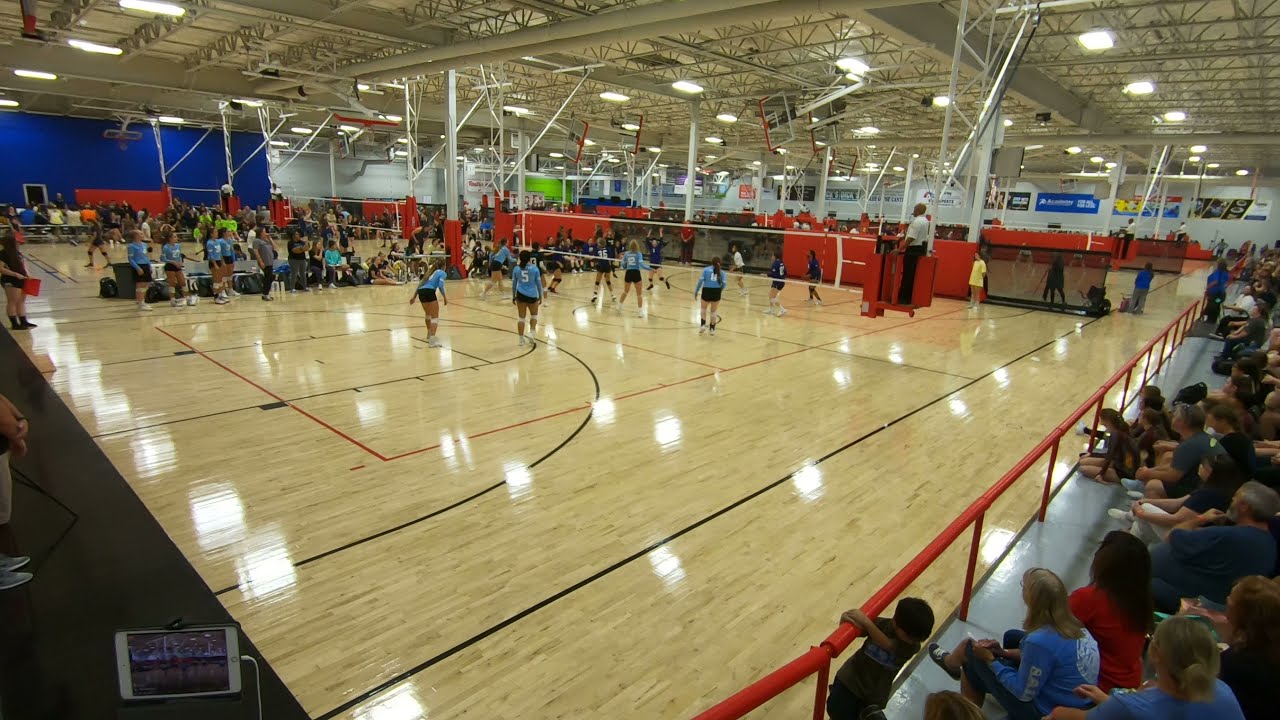This bright photo captures the energetic atmosphere of a women's volleyball game inside a spacious gymnasium. The gym features a shiny, tan-colored wood floor adorned with red and black stripes marking various sections of the courts. In the center of the image, a volleyball net with white borders and black netting stretches across the court, with a referee stationed in an elevated position for a better vantage point.

The team in the foreground, identifiable by their black shorts and blue t-shirts, are actively engaged in the game. One player, prominently wearing the number five, stands out among her teammates. To the right, the opposing team sports darker jerseys, possibly dark purple, though the exact color is somewhat difficult to discern.

Surrounding the court, walls painted in blue and white, along with some signage in the background, frame the space. A crowd of spectators, comprising men, women, and children, watches the game with keen interest from behind a red metal guardrail. The seating area includes individuals standing and sitting, some even leaning on the railing, fully immersed in the action and excitement of the volleyball matches taking place in the expansive gymnasium.